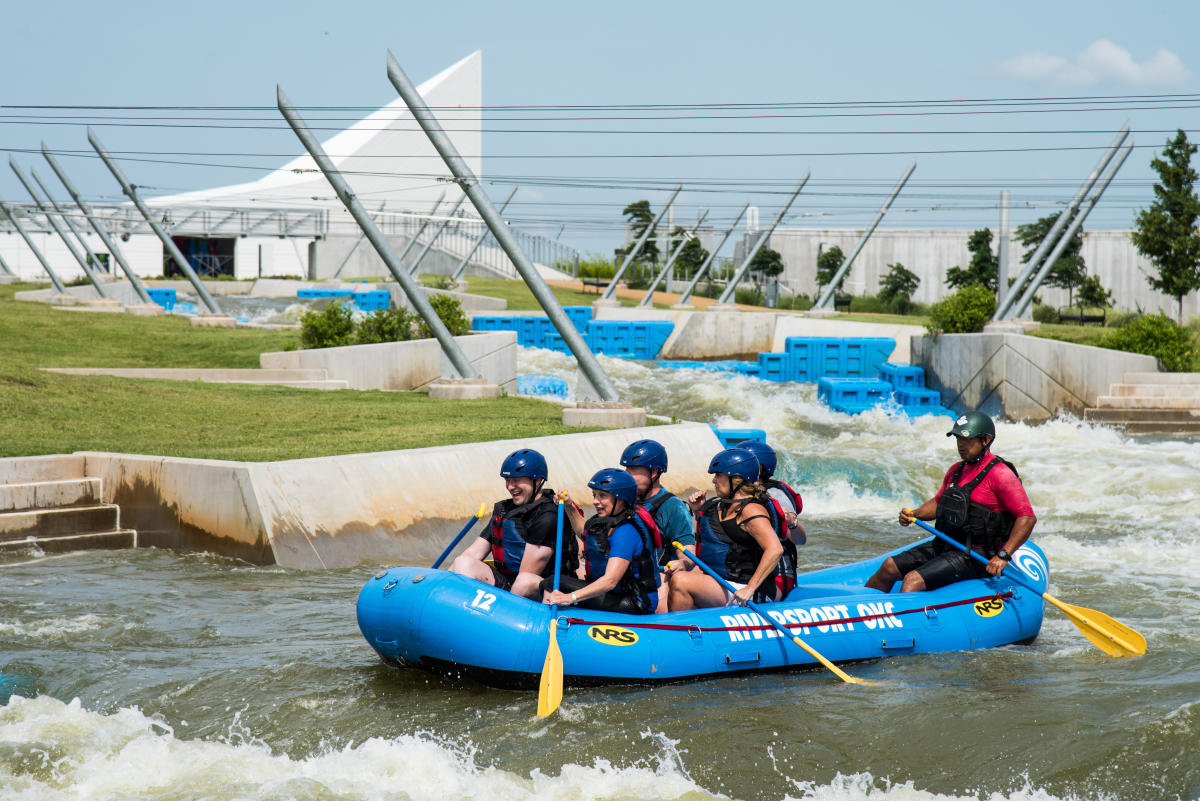In this rectangular vintage-style photograph, six people are aboard a blue raft navigating through rapid waters, giving the image a dynamic and exhilarating feel. The scene is reminiscent of the 1980s, characterized by its nostalgic color palette. The group appears to be engaged in a white-water rafting adventure, likely facilitated by a rafting company, as suggested by the steps leading down into the water which might serve as a launch point.

In the front of the raft, two individuals hold blue oars with yellow paddles, ready to steer through the challenging currents. Behind them, two more individuals are seated in the second row, also gripping their oars with determination. A solitary rafter is positioned in the third row, seemingly focused on the rush of the rapids. At the rear of the raft, separated slightly from the others, is the guide or navigator, who appears experienced and in control of the vessel.

The side of the raft is marked with “River Sport OKC” in white print, indicating the name of the rafting company. Additionally, the number '12', also in white print, is visible at the front, likely identifying the specific raft. It's a clear, daytime image, capturing the expressions of excitement and adventure on everyone's faces as they embrace the thrilling ride.